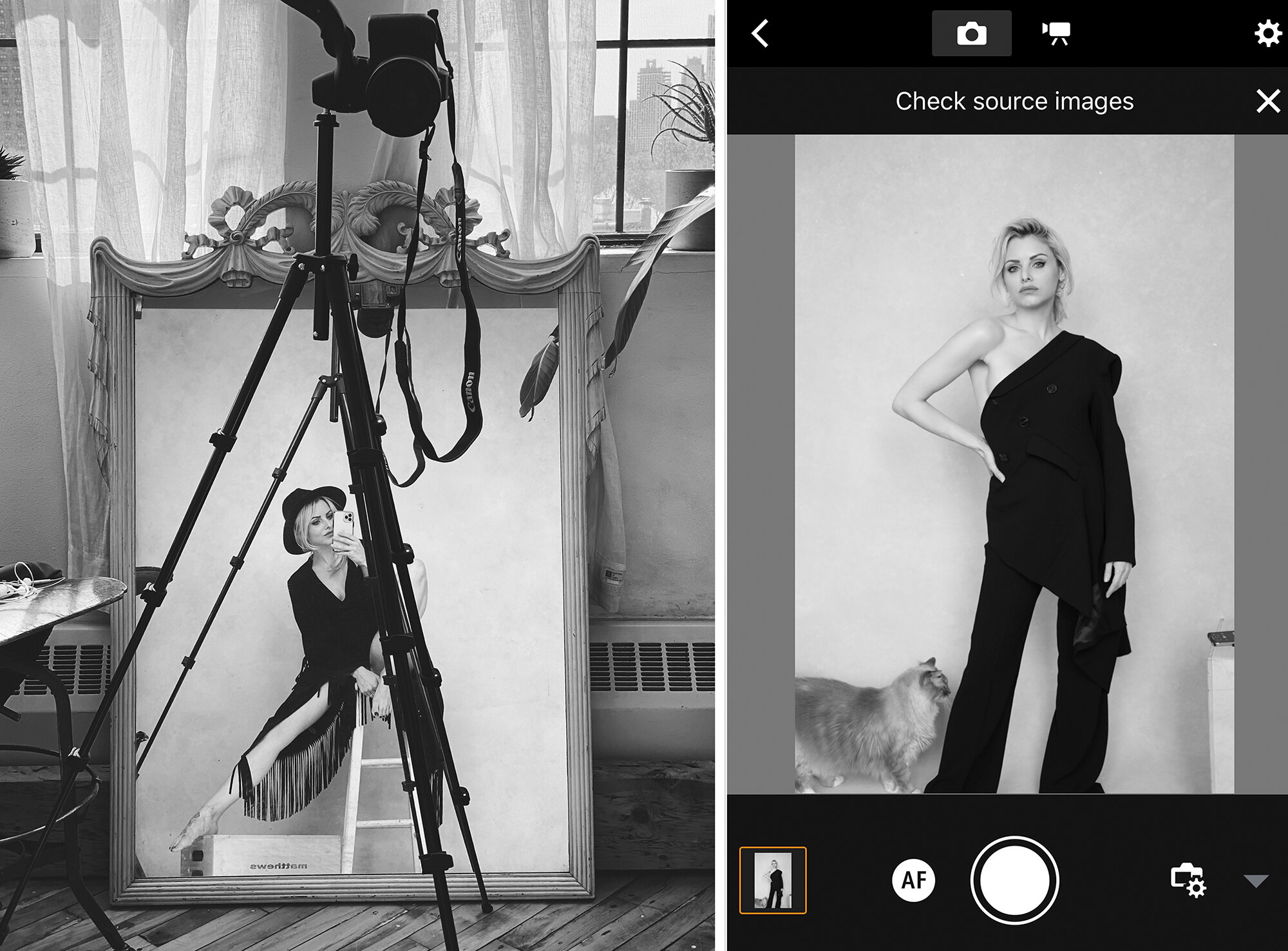The image depicts two monochromatic side-by-side photographs featuring the same blonde woman. In the right image, she stands confidently with one arm on her hip, dressed in a stylish asymmetrical black pantsuit with one sleeve on and the other off, accompanied by a long-haired cat at her feet. This setting resembles a digital camera interface, complete with dials, buttons, and a "check source images" prompt on the screen. On the left side, the woman is seated on a stool, striking a pose in a black fringed flapper-style dress and a black hat. She appears to be preparing to take a selfie, holding an iPhone while a professional camera on a tripod stands before her, placed against a backdrop of a room with elaborate decor, including an ornate mirror, sheer-curtained windows, and visible city buildings outside. The imagery showcases a blend of vintage style with modern technology, capturing moments of poised self-expression and creative self-portraiture.